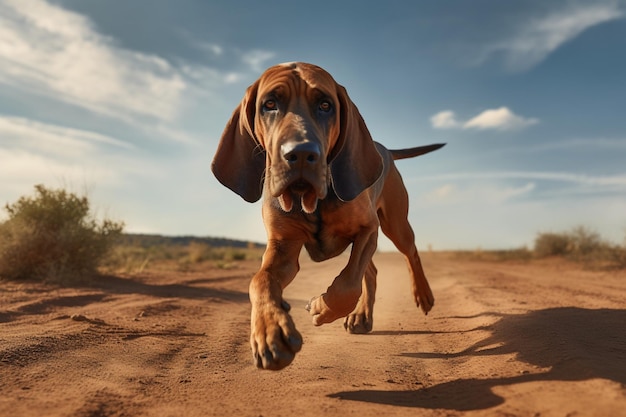The image is a horizontal landscape photograph taken outdoors in the countryside during the daytime under a sunny sky, adorned by a few white, wispy clouds primarily in the top left-hand corner. The scene features a bloodhound running dynamically towards the photographer along a barren, dry dirt path. The dog's brown coat is highlighted with subtle black markings on its back and around its eyes. Its prominent, floppy ears, saggy cheeks, and extended tail add to its expressive mid-trot posture, with three of its legs suspended in the air and the back left leg just touching the ground. A shadow of the bloodhound is clearly cast on the bottom right corner of the image, indicating that the sunlight is coming from the top left. Flanking the dusty trail are small, sparse bushes located on the mid-left and mid-right edges of the frame, adding a touch of greenery to the predominantly earthy landscape.